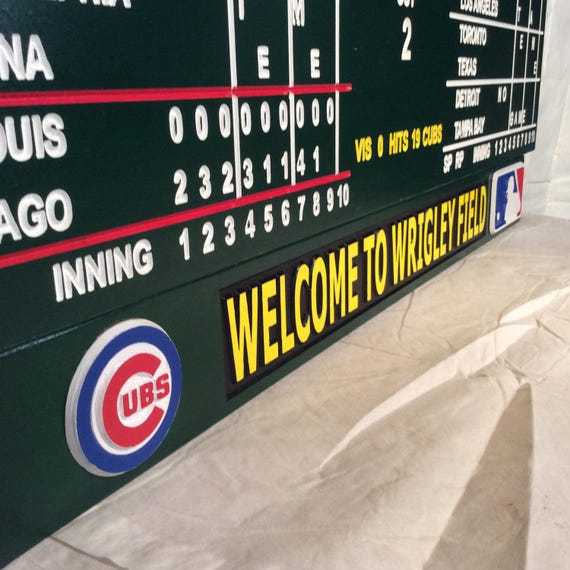This image features a meticulously detailed, decorative replica of the historic Wrigley Field scoreboard, known for being home to the Chicago Cubs. The scoreboard is crafted from wood, painted in dark green, and displays carved-in scores and details, suggesting it is not a functional, manually-operated scoreboard. Positioned on a tan marble counter, accented with streaks of white and gray, the board appears well-lit and located inside an indoor setting, possibly a sports room or bar.

At the bottom left, the iconic Cubs logo is prominently displayed, consisting of a large red "C" with "UBS" nestled inside, against a white background surrounded by a blue circle. Adjacent to this, in bold yellow text over a black bar, the phrase "Welcome to Wrigley Field" offers a warm greeting, accompanied by the Major League Baseball (MLB) logo on the bottom right. The MLB logo features a silhouette of a batter against a blue and red backdrop with a white stripe.

The upper sections of the scoreboard list various baseball game scores in white text. The main score area highlights the innings from 1 to 10, showing detailed match results with Chicago competing with St. Louis. Chicago's team has impressive innings scores reflecting 2, 3, 2, 3, 1, 1, and 4, totaling 19 hits, while St. Louis has a string of zeros. Additional sections of the board feature statistics of other games, partially visible with team names such as Los Angeles, Toronto, Detroit, and Texas.

Despite the close-up angle cutting off some parts, the scoreboard's intricate design and historical references to Wrigley Field triumphantly capture the grandeur and nostalgic charm of Chicago Cubs baseball history.